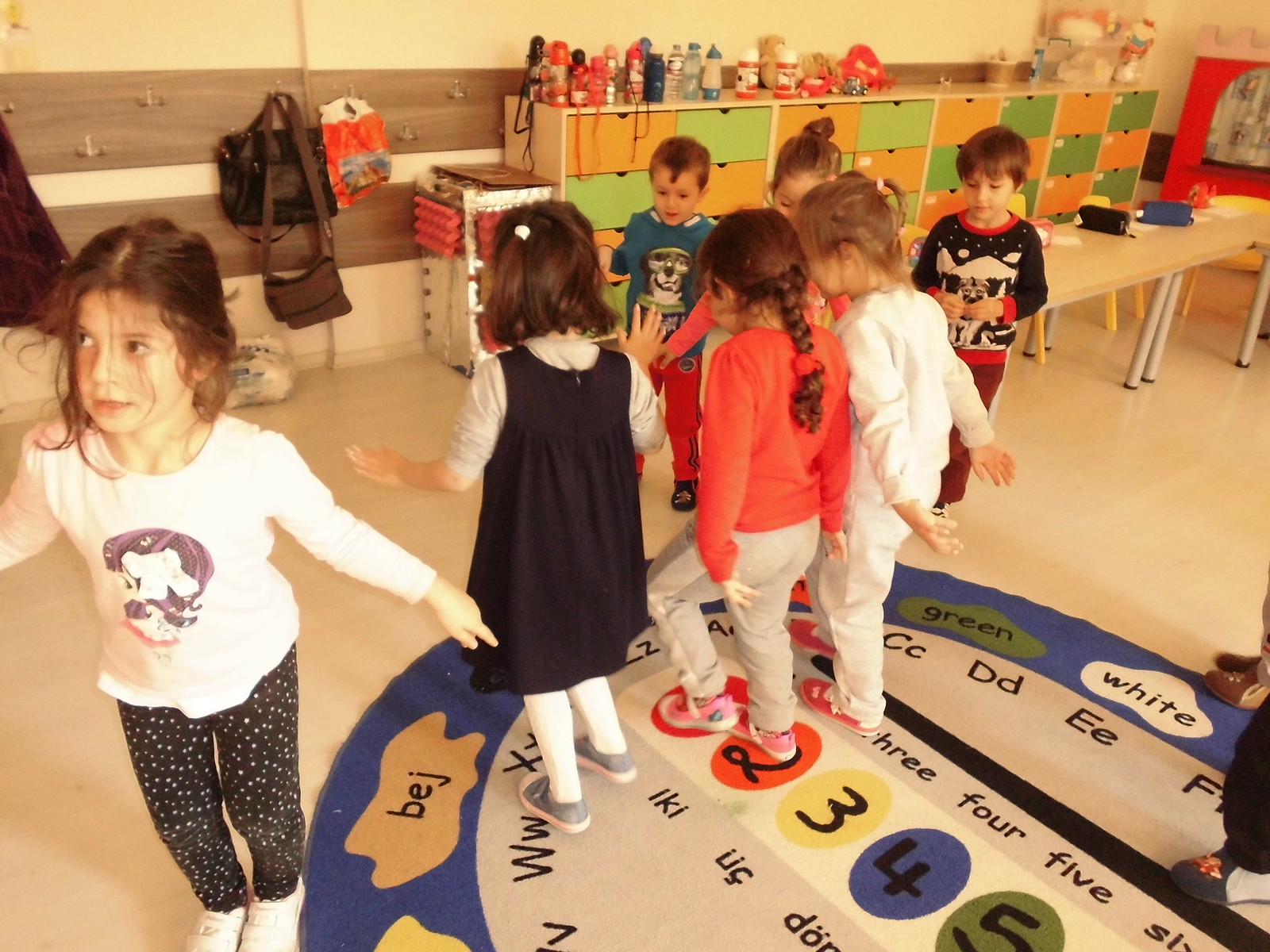In the photograph, a group of seven young children, likely 1st or 2nd graders, are gathered in a warmly lit, clean classroom. The children, approximately four or five years old, are engaging in an activity on a colorful mat positioned on the white laminated floor. The mat is decorated with various learning materials, including numbers (3, 4, 5, 6, 1, 2) in circles of varying colors (red, yellow, blue, green), and letters spelling out numbers and colors.

To the left, a little girl stands out prominently. She is wearing a My Little Pony shirt, black and white speckled pants, and white shoes, and her long hair is tied back. She is looking up towards the corner of the image, capturing a sense of curiosity. Surrounding her are three more girls facing away from the viewer, while two boys and a girl stand opposite them.

The classroom features a back wall painted in cream and brown. Against this wall is a storage unit with green and orange sections, topped with an array of colorful water bottles. Hooks for hanging backpacks are visible on the left side of the image, with a couple of bags already in place. In front of the storage cubbies, there are a few low tables with steel legs and wooden tops, laden with various study materials. The overall atmosphere feels organized and conducive to learning.